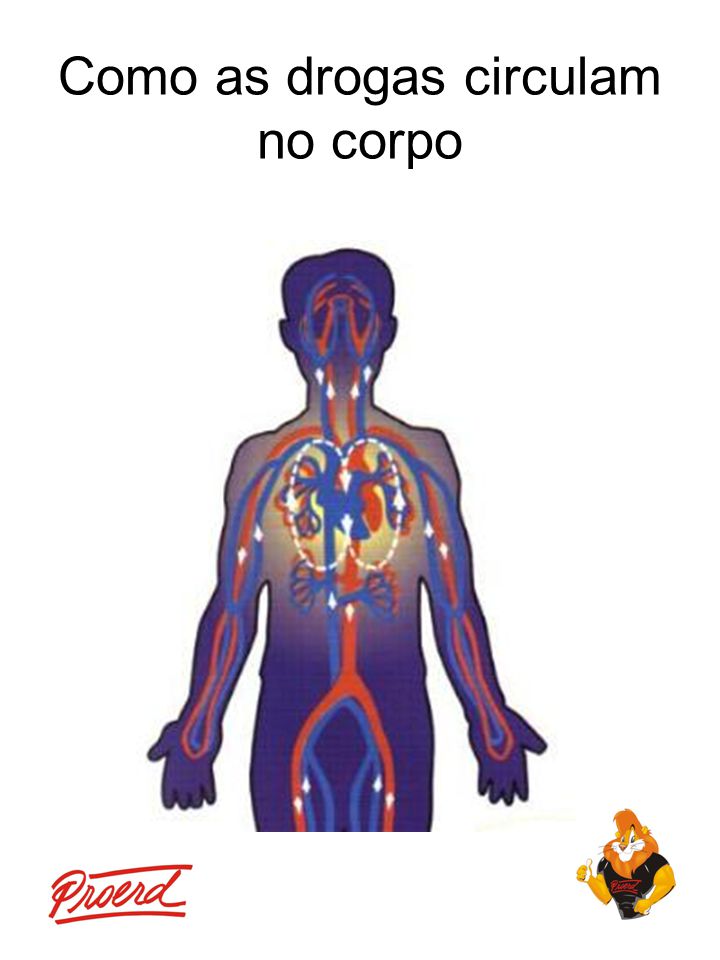This is an educational image showcasing an outline of a human body's circulatory system. The top of the image features black text in a foreign language, likely Spanish, with the phrase "como es drogas circulam no corpo." Below this, there is a simple, animated silhouette of a person, predominantly shaded in a purplish-blue hue. Around the heart and lung area, the coloring transitions to yellow. The circulatory system is depicted with blue veins and red arteries, extending to the head, arms, and legs, showing the blood flow with arrows and dotted lines. The lungs and kidneys are noticeably included in the rough outline. At the bottom left corner, there's red cursive handwriting that reads "poerd" or possibly "pro-word." In the lower right corner, a cartoon lion with an orange mane and a black t-shirt gives a thumbs-up, adding a whimsical touch to the otherwise educational illustration.